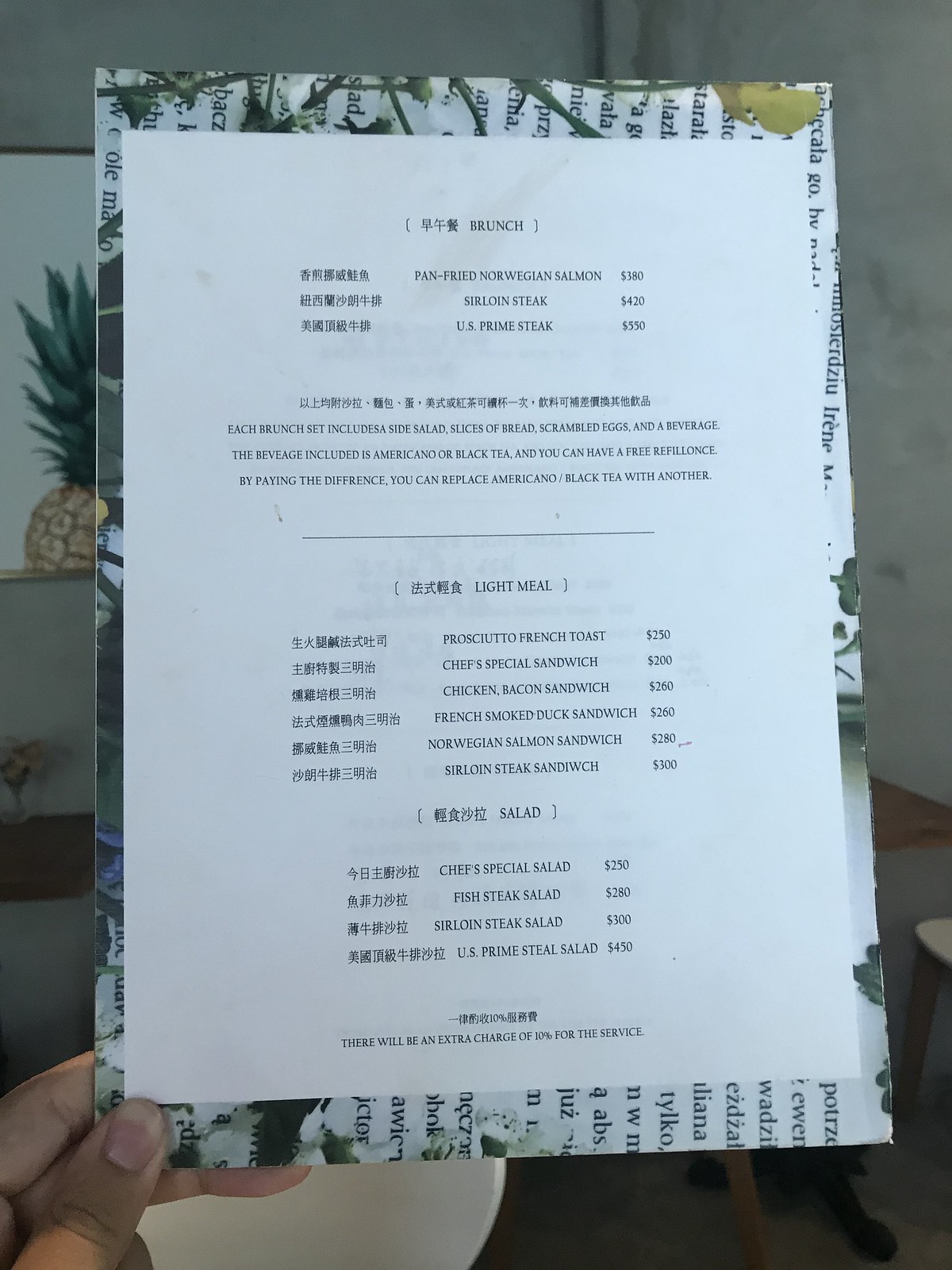The photograph captures a close-up view of a menu being held by a person's left hand, which is visible emerging from the bottom left side of the image. The thumb, middle, and index fingers are distinctly seen, along with the knuckle of the right thumb just peeking out at the edge of the frame. Beneath the hand, there is a white circular object, possibly a plate, partly visible. The background showcases a table, providing a stable surface beneath the menu.

The menu itself has a decorative border, resembling another menu design, adorned with plant-like branch motifs adding a touch of elegance. The menu text is bilingual, presented in both English and Chinese. Divided into sections, the menu's top part is titled "Brunch," followed by a "Light Meal" section, and concluded with a "Salad" section at the bottom.